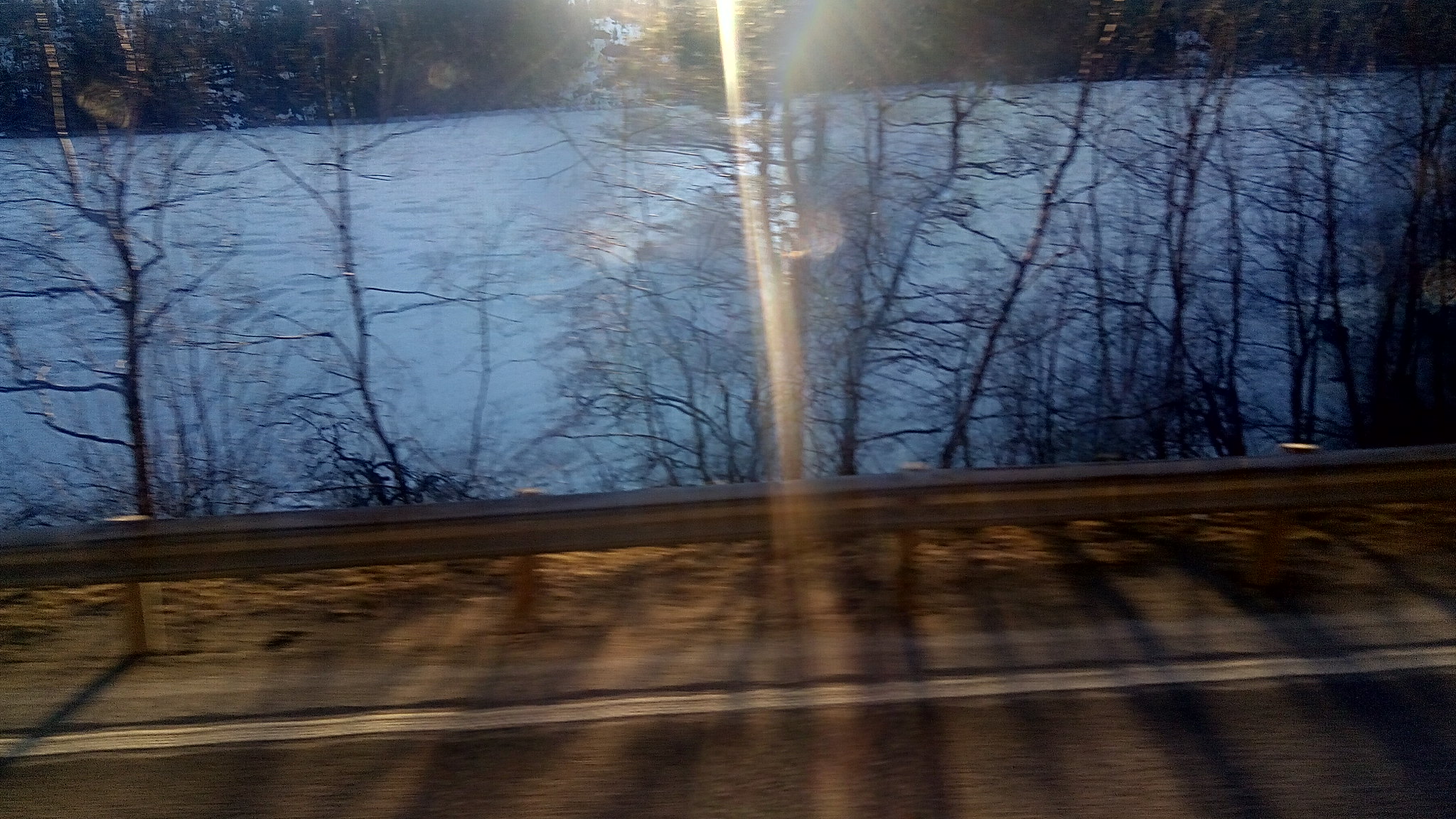This photograph captures a slightly blurred image of a lakeside scene, likely taken from a moving vehicle. The bottom of the image shows a stretch of asphalt road with a visible white line and a gray metal guardrail. A mix of dirt and patches of snow can be seen beyond the guardrail, indicating wintertime as the trees are bare with no leaves. In the distance, a dark, tranquil lake is framed by wooded areas on either side. The sky is relatively dark, suggesting it is either sunrise or sunset, with a soft halo of light near the horizon and faint rays in the top center of the image. Overall, the image portrays a quiet, wintry countryside moment with a somewhat ethereal quality due to the natural light and motion blur effect.